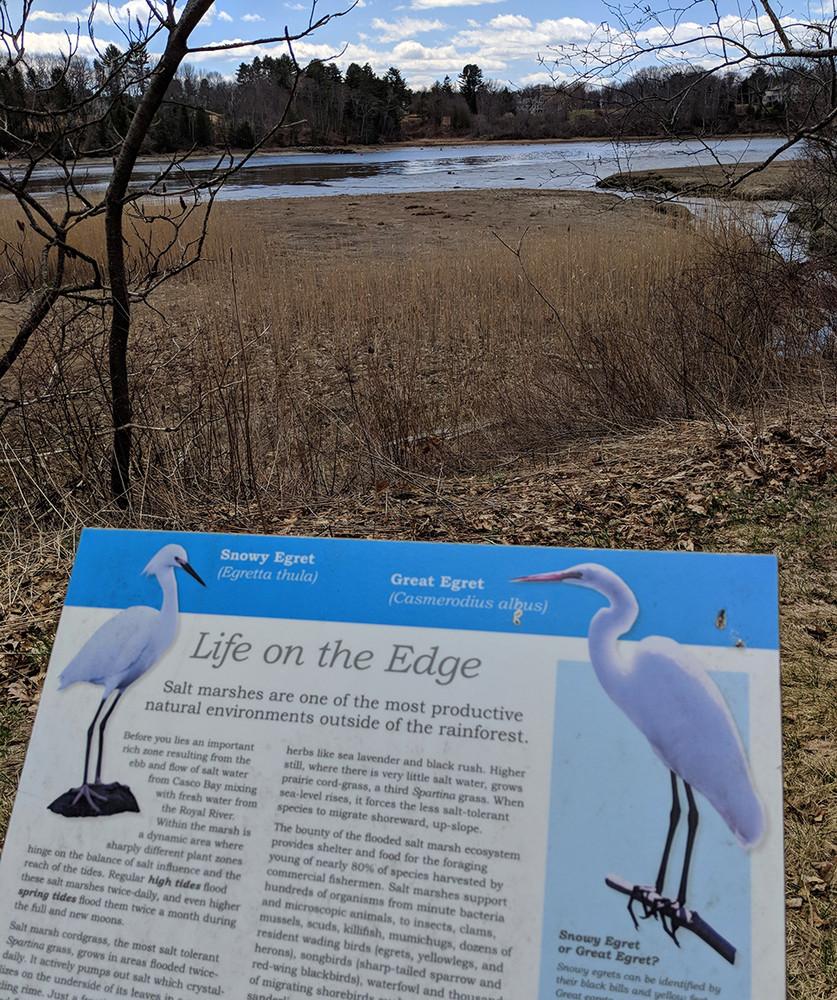The photograph captures a picturesque scene, possibly within a nature reserve or park, where a sign titled "Life on the Edge" stands prominently in the foreground. The sign features detailed images of two birds: a snowy egret on the left, and a great egret on the right, both native to the marshland depicted. The snowy egret is illustrated as a white bird with long legs, while the great egret is similarly white, characterized by an orange beak and black long legs. Below the images, the sign provides extensive information about the importance of preserving salt marshes, one of the most productive natural environments outside of the rainforest.

In the background, a tranquil stream meanders through a varied landscape of trees, with tall pines and other deciduous trees, some barren and others adorned in greenery. The marsh grass appears brown and tall, indicating a somewhat dried-up state, while the stream itself is murky blue. The sky overhead is a bright, light blue filled with numerous fluffy white clouds, suggesting a sunny day. The scene showcases the natural habitat that these egrets and other wildlife rely on, emphasizing the delicate balance of life on the edge of the marshes.